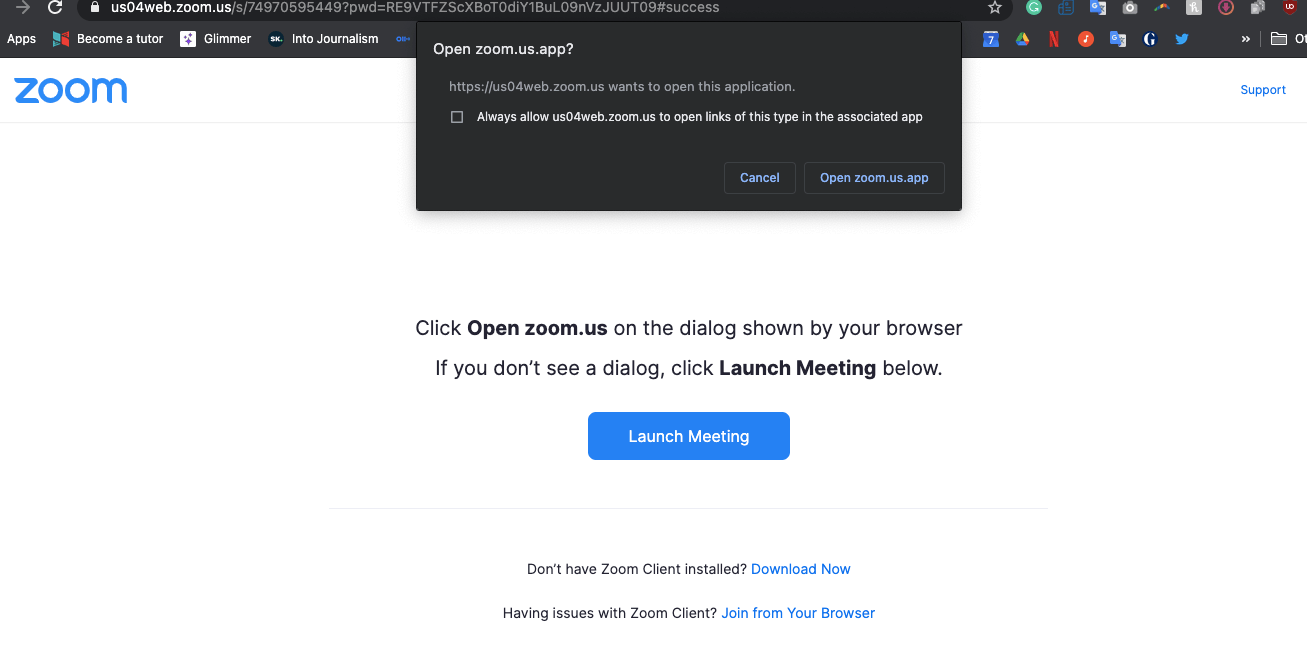The screen displays an active Zoom meeting interface. At the top, a right arrow, followed by a refresh icon, is visible. The URL "us04web.zoom.us?s=7497055449&pwd=RE9VTFZSCXBOT0DIY1BUL09NVZJUUT09#success" is prominently featured. Below this, a series of application icons are displayed, including a holostar, the Grammarly icon, a blue unidentified icon, Google Translate, a camera icon, a rainbow-colored Boomerang, and a red microphone. 

The interface also contains a text bar labeled "Apps" on the left side, alongside a label "Blue Left" and an option to "Become a Tutor." Additionally, a glamour icon with a sparkly effect labeled "Antigenism" is centered prominently. 

At the top, larger squares represent the "Open Zoom.us.app" option, requesting permission to "Always allow us04web.zoom.video to open links of this type," with "Cancel" and "Open" buttons available. 

Other icons displayed include Google Drive, Netflix, music apps, Google Trends, Instagram (IG), Twitter, and Support. There is also a message indicating instructions to "Click open zoom.us," explaining that dialogs should appear in the browser and offering the option "If you don't see the dialog, click launch menu below." The launch menu icon appears with the note "Don't have Zoom client?"